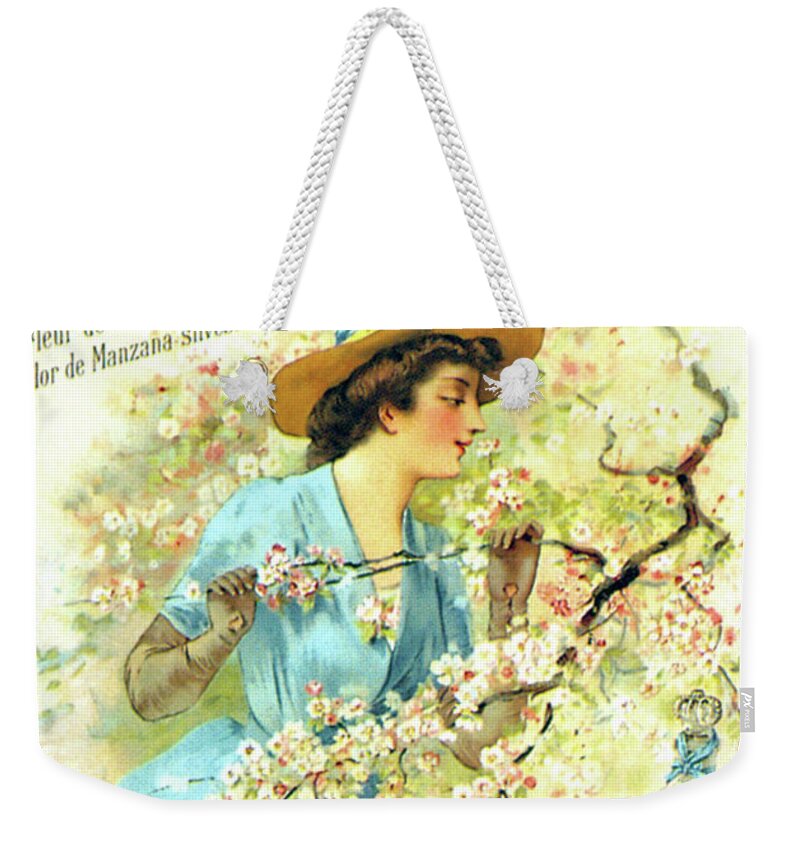The image showcases a canvas tote bag adorned with a detailed reproduction of an 1800s painting or illustration. The design depicts a young white woman with curly brown hair, dressed in a flared blue dress and long gray gloves. She is wearing a straw gardening hat that shields her from the sun. Engrossed in the beauty of a flowering tree, possibly a cherry blossom, the woman gently holds and inspects a branch covered in clusters of pink and white flowers. Her rosy cheeks suggest delight as she admires the blossoms, looking to her left, which is the right side of the bag from our perspective. In the top left corner of the image, there is partially visible text, with the words "de manzana" discernible. The tote bag features a practical twine or woven cloth strap, contrasting with its artistic and historical design.